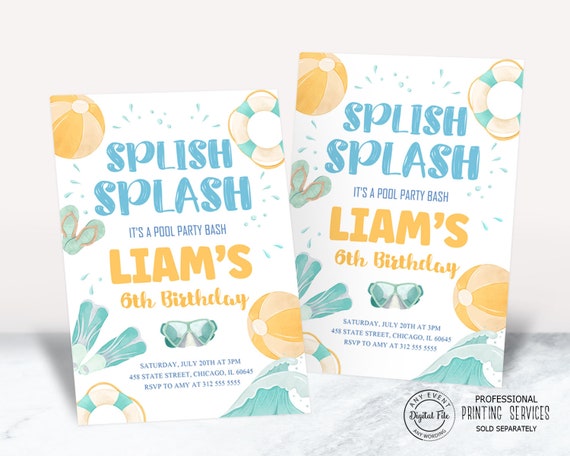This image is a promotional photograph for a printing service that specializes in creating party invitations. The scene features two identical birthday invitation cards set against a white or off-white backdrop with a grayish marble counter underneath. In the bottom right corner of the image, there's a watermark indicating professional printing services are sold separately, and any event digital file can have any wording.

The invitation cards prominently display text in festive fonts and vibrant colors. At the top, light blue text reads "Splish Splash." Beneath that, smaller text states, "It's a Pool Party Bash," followed by bold yellow text announcing "Liam's Sixth Birthday." The event details in dark blue text at the bottom inform guests of a party on "Saturday, July 20th at 3 p.m., 458th State Street, Chicago, Illinois, 60645," and include RSVP details: "RSVP to Amy at 312-555-5555."

Decorating the borders of the cards are cheerful illustrations of beach-related items. There are orange and white beach balls in the top corners, orange and green lifesaver floaties in the right and bottom left corners, and various other summery graphics like ocean waves, slipper flippers, and sandals. The overall color theme of the invitations includes splashes of yellow, light blue, teal, and a touch of tan, giving them a playful and inviting look perfect for a pool party bash.